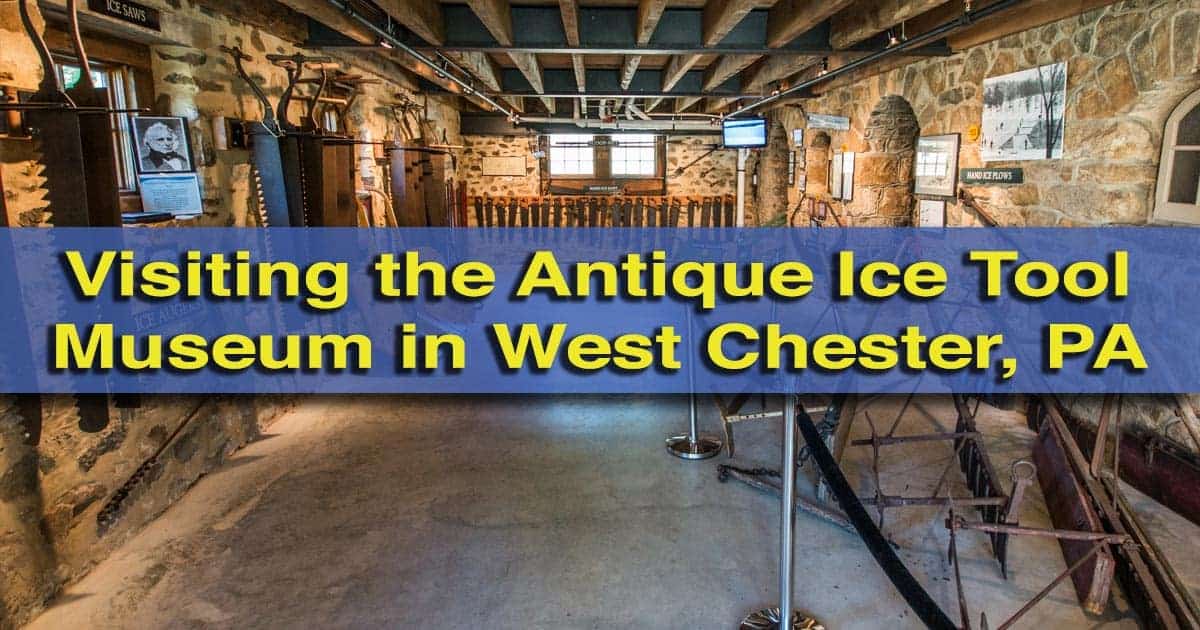In the image, a blue translucent horizontal strip with 3D yellow text reading "Visiting the Antique Ice Tool Museum in West Chester, PA" stands prominently in the middle. The background features an interior photograph of a museum room with irregularly shaped brown brick walls adorned with various paintings and posters. The room has flat, gray floors and a ceiling supported by brown wooden logs and beams. The overall space appears to be rectangular in shape, with different objects placed near the walls, and some pipes crossing the ceiling, contributing to a rustic, cluttered ambiance.